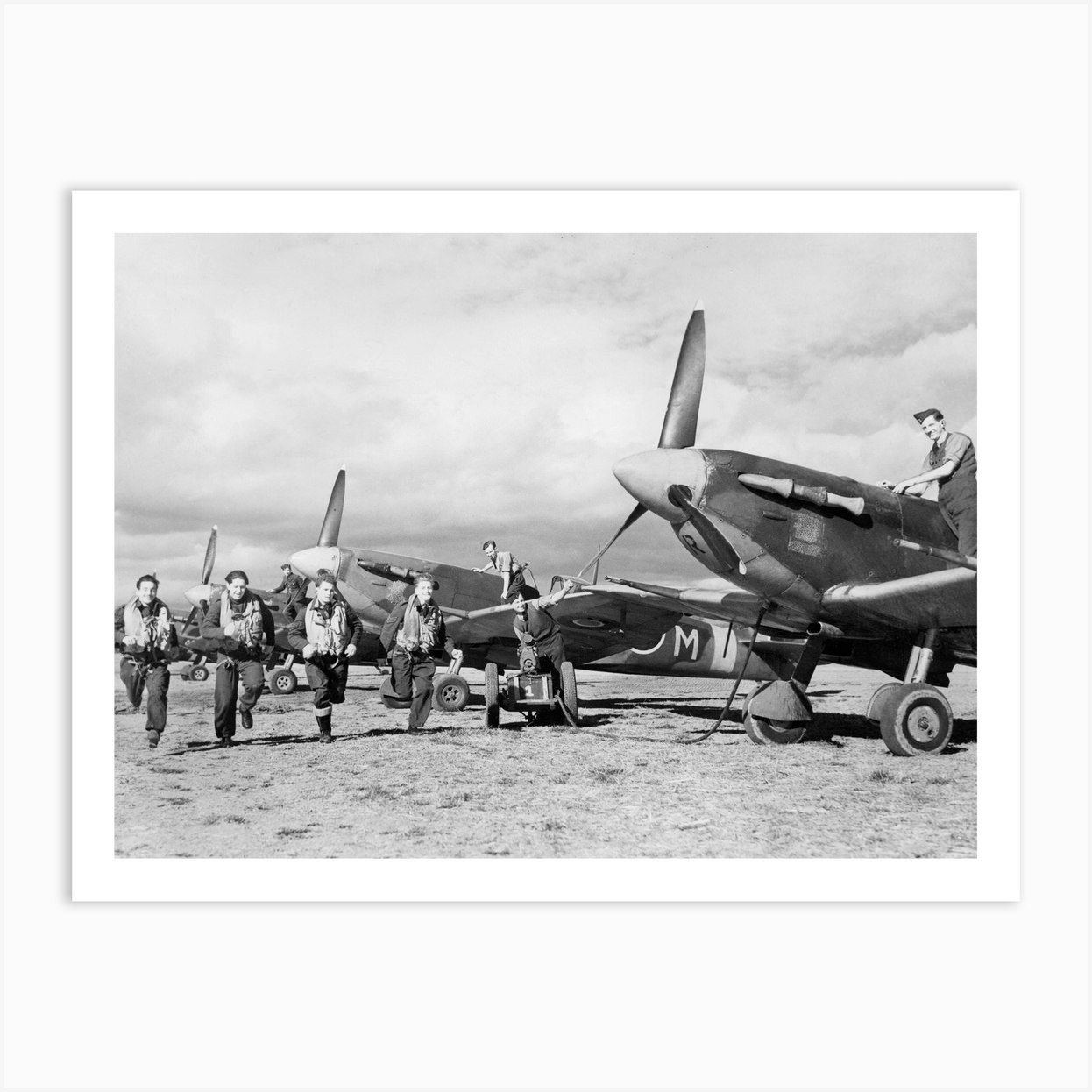This black and white photograph, centrally positioned within a perfectly square frame with a white background, captures a dynamic scene set against a backdrop of overcast skies. Four Caucasian men, sporting light-colored vests paired with dark long sleeves and pants, are seen running across a grassy field amidst a row of stationary, old-model propeller airplanes. Among the aircraft, two men are engaged in maintenance—one atop an airplane and another on the ground beside a running man using a small Segway-like device. Shadows cast by the men suggest intermittent sunlight filtering through the clouds. The overall ambiance and gear hint at a military setting, embodying a sense of urgency and purpose.